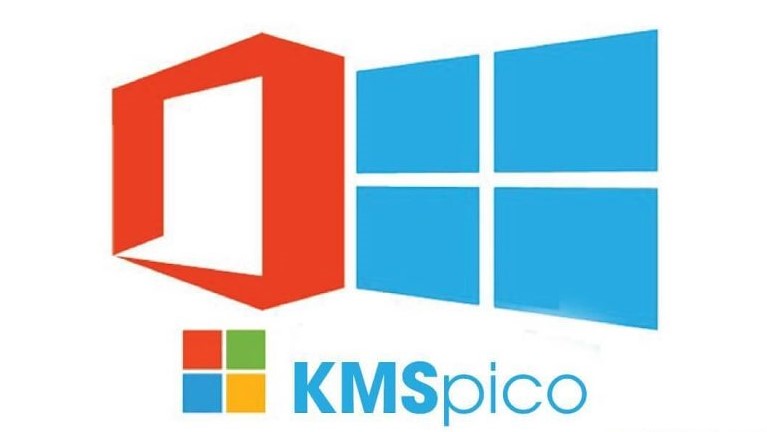The image features a company logo on an all-white background. On the left side of the logo, there is a red cube with a white interior. Adjacent to the cube are four blue rectangles arranged vertically. Below these rectangles, there is a smaller set of four squares in different colors: red, green, blue, and yellow. To the right of these shapes, in blue lettering, are the words "KMS" in larger font and "PICO" in smaller font directly underneath. The placement and variety of shapes and colors suggest a stylized representation, possibly relating to different versions of Windows logos. This cohesive arrangement of distinct geometric elements and text forms a unified and visually engaging design in the center of the image.